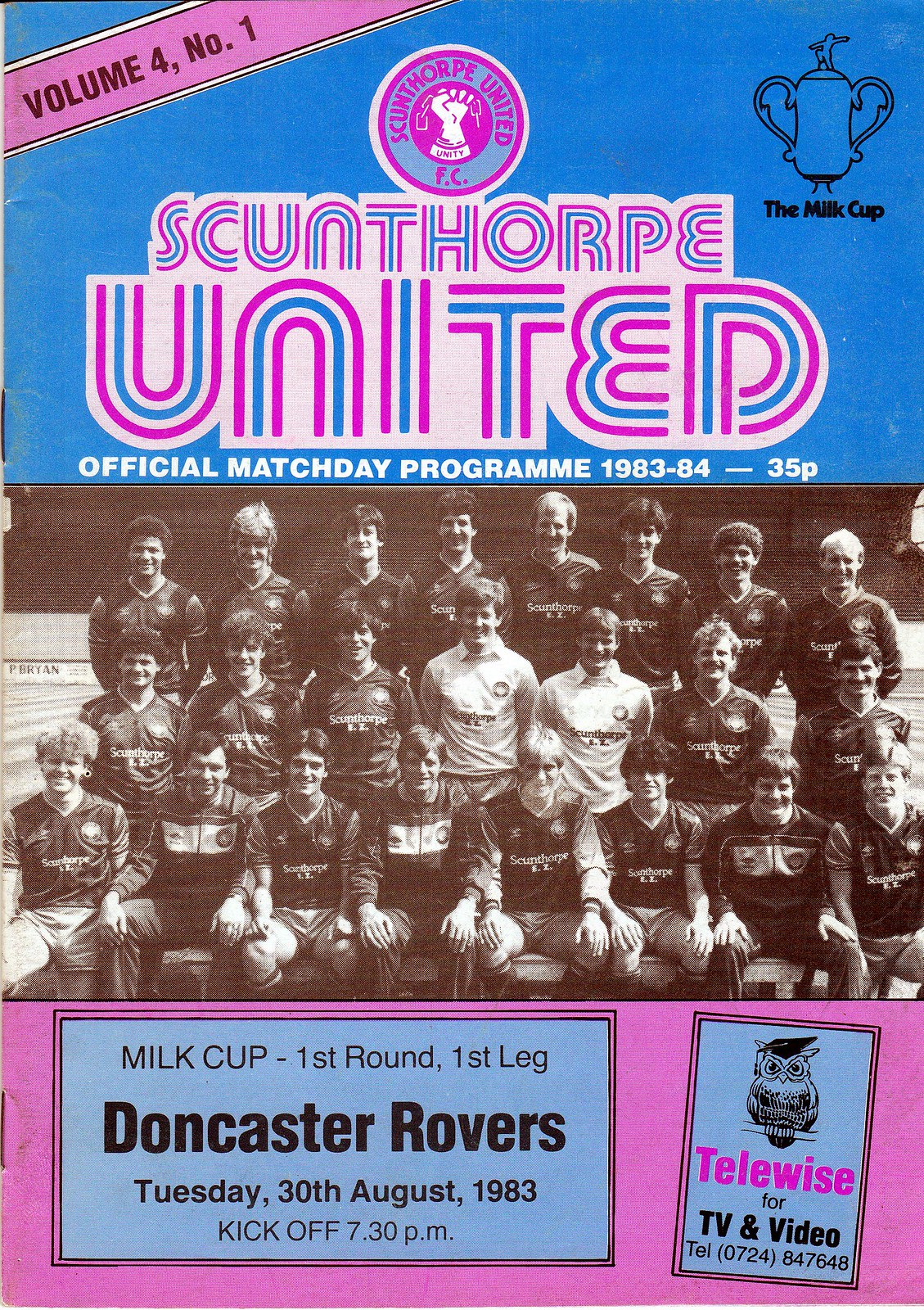This image is the cover of an official Match Day program for Scunthorpe United FC, dated Tuesday, 30th August, 1983. The top third of the cover is blue, featuring a pink ribbon across the top left that reads "Volume 4, Number 1." Across the top, the text "Scunthorpe United" is prominently displayed in blue and pink with a white border, resembling neon lights. 

Central to the cover, there is a black-and-white photo of the Scunthorpe United soccer team. The team is arranged in three rows: the front row seated on the ground, the middle seated on chairs, and the back row standing. Below the team photo, in black letters on a blue background, it reads "Milk Cup, First Round, First Leg, Doncaster Rovers, Tuesday, 30th August 1983, Kickoff 7.30PM." 

On the right side of the image, there's an advertisement for Telewise showcasing a black owl with a graduation cap, accompanied by the text "Telewise" in pink letters and a contact number "(0724) 847648" in black letters on a blue background. The background of this section is pink. Additionally, the cover highlights this being the "Official Match Day Program 1983-84" and the cost of "35p" in white letters on a blue background.